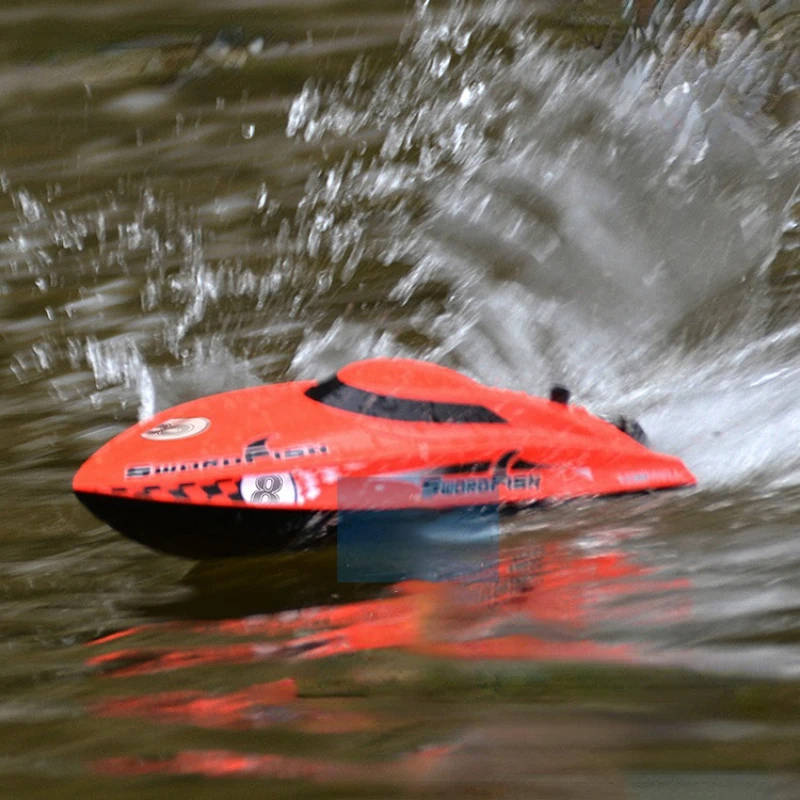This color photograph captures a blurred, dynamic scene of a red toy speedboat racing across murky, rippled water. The speedboat is completely enclosed with no visible occupants and features black and white graphics, including a checkered pattern and a prominently displayed "Swordfish" label on the side. It also has a black and white windshield with deep, dark tinted panes. As the boat speeds through the water, it kicks up a huge splash behind it, with droplets appearing disproportionately large, suggesting it's a remote-controlled model. The background and foreground are composed entirely of water, adding to the impression of high velocity and action captured in the image. Additionally, there is an overlapping gray rectangle, resembling a watermark, in the lower center of the photo. The craft has various decals, including advocacy ribbons and emblems that contribute to its race-like appearance. Despite the blurriness, the boat’s vibrant red color and detailed graphics are striking against the muted tones of the surrounding water.